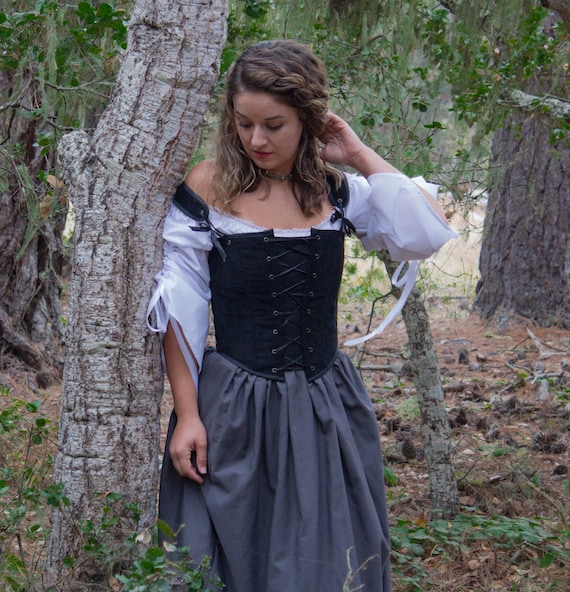In this image, a young brunette woman is captured in a serene, forested setting, surrounded by several large tree trunks and lush greenery. She's dressed in a Victorian-style ensemble, featuring a black corset paired with a gray skirt, and white sleeves accentuating her outfit. Her curly shoulder-length brown hair is styled with a loose braid sweeping across her forehead. The woman is standing straight, leaning her right shoulder against one of the large tree trunks, her posture composed with one hand elevated to touch her hair and the other resting at her waist. She gazes downward, contributing to the muted, contemplative atmosphere of the scene.